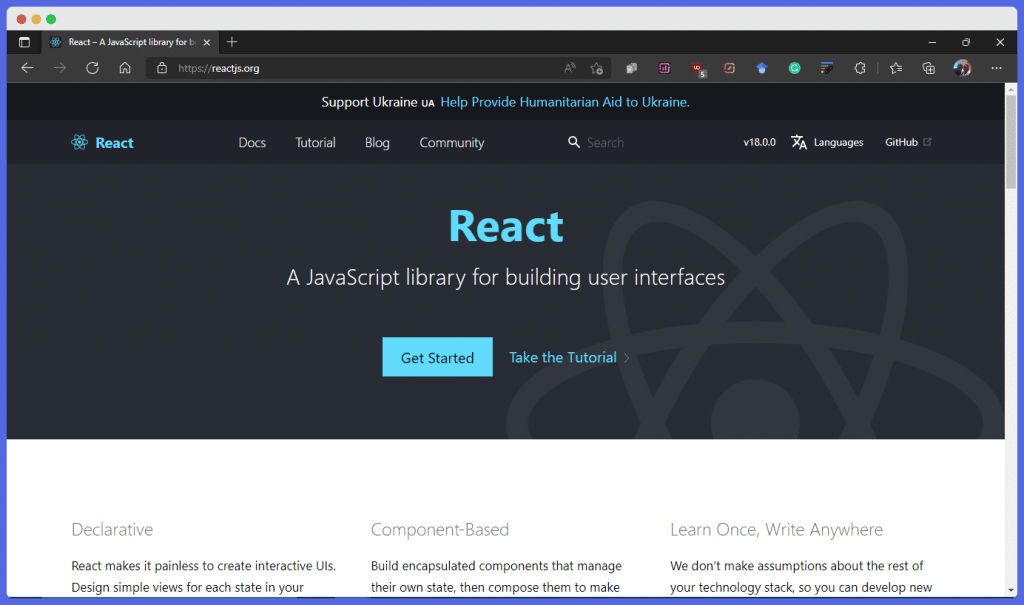Screenshot of the ReactJS Homepage Displayed on Chrome with Dark Theme on a Mac

This screenshot showcases the ReactJS website (reactjs.org) viewed on a Chrome browser with a dark theme, most likely on a Mac, as indicated by the presence of the distinctive stoplight buttons (red, yellow, and green) on the top-left corner of the window.

The browser tab displays the text "React - A JavaScript library for," truncated before it completes. At the top banner of the website, a black rectangle with white text reads "Support Ukraine, UA," accompanied by a blue hyperlink saying "Help provide humanitarian aid to Ukraine."

The main menu bar, a dark gray rectangle, features the React logo—rendered in blue with an intricately outlined mandala-like pattern. The navigation items in white font include "Docs," "Tutorial," "Blog," and "Community." Additionally, there is a search function represented by a white-outlined magnifying glass icon, with the word "Search" in gray, followed by the version number "V18.00," a language translation dropdown labeled "Languages," and an external link to GitHub.

Central to the webpage, the React logo appears again in a large blue bold font, accompanied by the tagline in gray font: "A JavaScript library for building user interfaces." Below this, a blue button labeled "Get Started" and a tutorial link titled "Take the Tutorial" featuring a right-pointing arrow are visible.

Towards the bottom of the page, three columns summarize React's core principles:
1. **Declarative**: "React makes it painless to create interactive UIs. Find simple views for each state in your."
2. **Component-Based**: "Build encapsulated components that manage their own state, then compose them to make."
3. **Learn Once, Write Anywhere**: "We don't make assumptions about the rest of your technology stack, so you can develop new."

The screenshot captures the essence of the ReactJS homepage, providing insights into its layout, content, and design elements.